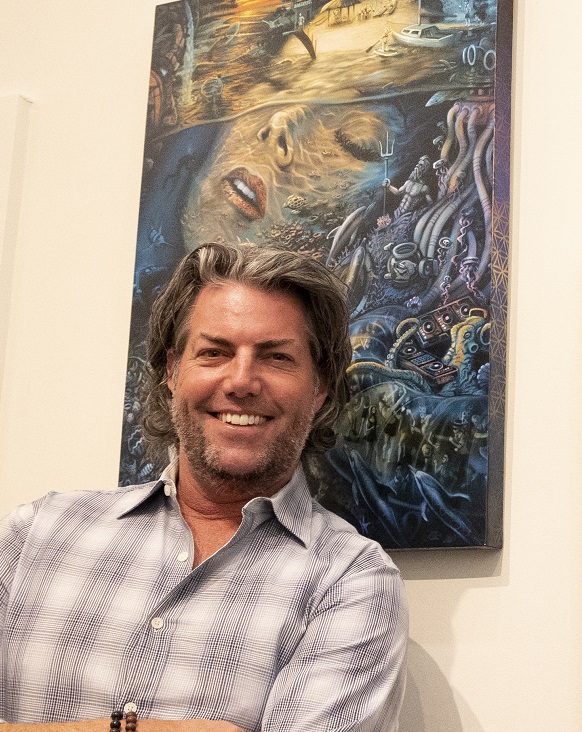A contemporary photograph features a man, likely the artist, smiling warmly in the foreground. He has graying, slicked-back hair and light skin, with patchy facial hair. He seems to be in his late 30s to mid-40s. He's dressed in a gray and white plaid button-down collared shirt with white buttons, and he's wearing two beaded bracelets—one brown and one black—on his wrist. The backdrop of the image is a white wall adorned with a vibrant painting.

The painting behind him depicts a woman’s face immersed underwater. The woman has red lips and closed eyes, set within a surreal, almost abstract underwater environment. Various vibrant details enhance the scene, including cyan and dark blue hues around her eyes, black mascara on her eyelashes, and black eyebrows. Her surroundings feature an array of underwater elements like octopus tentacles in purple and blue shades, a small gray boat, various brown and cyan objects, vases, and even electronics like a phone. Additionally, mythical elements such as a statue resembling either King Triton or Poseidon, adding an intriguing narrative layer to the piece, are seen alongside other aquatic creatures like dolphins and corals. The overall painting is extremely colorful and filled with intricate, whimsical details that seem to merge the realms of reality and fantasy.